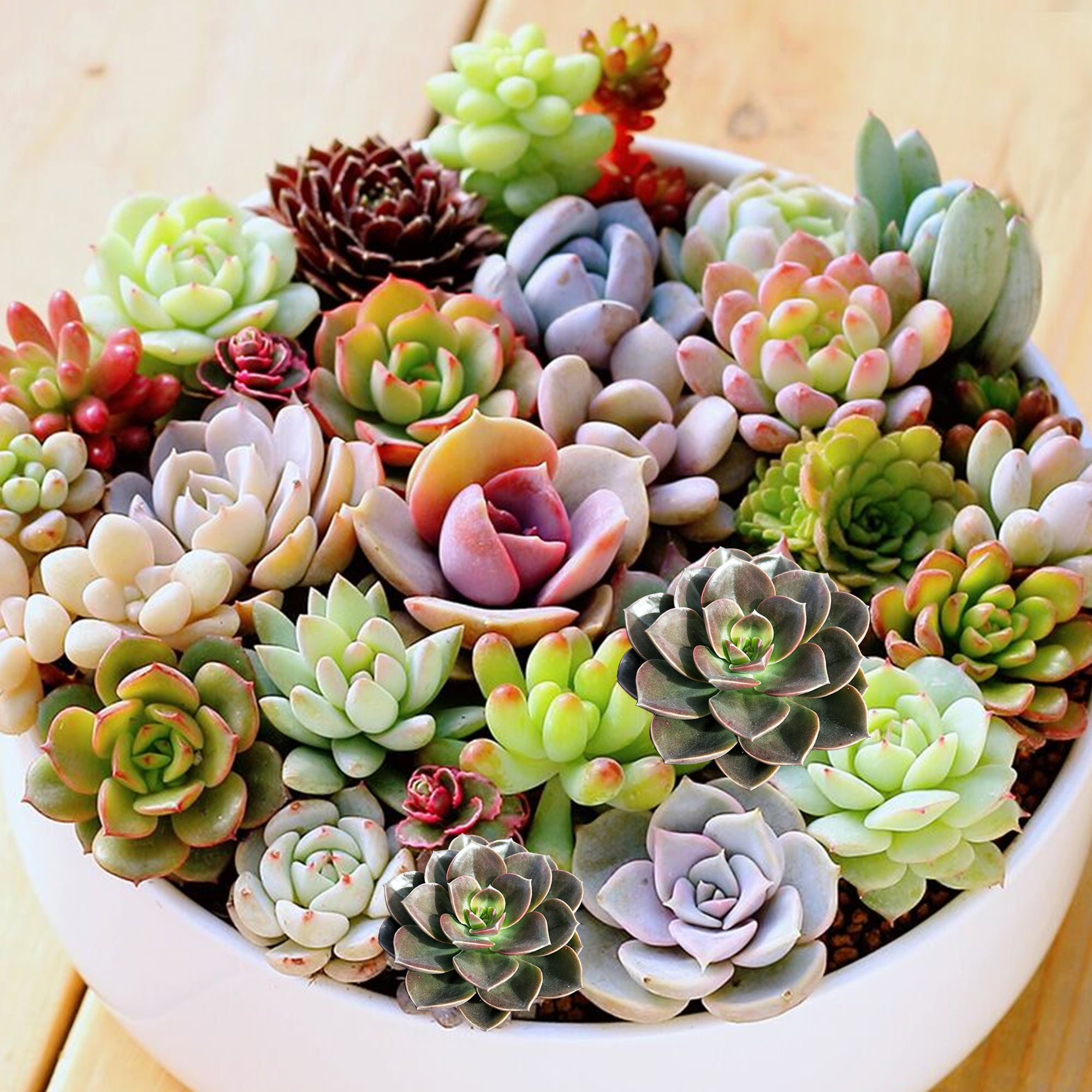The image features a large, round, white bowl, prominently placed on a light brown wooden table with noticeable horizontal slats. This cereal-sized bowl is brimming with an assortment of small flowers, possibly plastic, showcasing a vibrant palette of colors. The flowers range from various shades of green, including a striking radioactive green, to rich hues of pink, light purple, red, brown, auburn, white, and even touches of grayish-black near the tops of some flowers. The arrangement appears densely packed, with around 20 to 30 flowers giving the bowl a lush, full look. The close-up nature of the photograph ensures the details of the flowers and their vivid colors are clearly visible, while the background remains subtly out of focus.